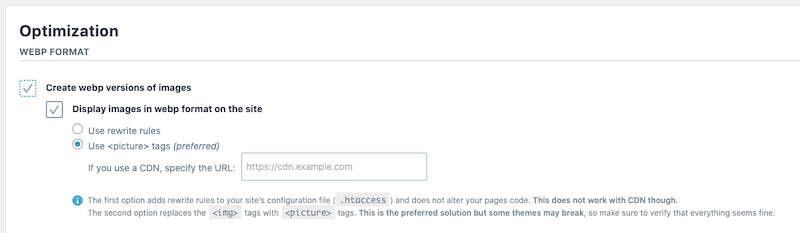This image displays a screenshot with a white background, bordered by a thin grey line on the upper and left edges. At the top left corner, the word "Optimization" is prominently featured in black, with a capitalized "O" followed by lowercase letters. Below this, in grey letters, it reads "WEBP format FORMAT." 

A thin grey line separates this title from the subsequent content. Immediately underneath, there is a square checkbox labeled "Create WebP versions of images," which is marked as checked. Indented below, another checked box reads "Display images in WebP format on the site." 

Further down, an indented grey circle with a white interior is labeled "Use re-write rules." Adjacent to this, a grey circle with a blue dot in the middle is labeled "Use picture tags (preferred)." 

Following these options, the text instructs, "If you use a CDN, specify a URL:" accompanied by a light grey-outlined text box for entering the website URL. 

At the bottom, a blue circle with a question mark provides additional context: "The first option adds re-write rules to your site's configuration file," followed by more detailed information.